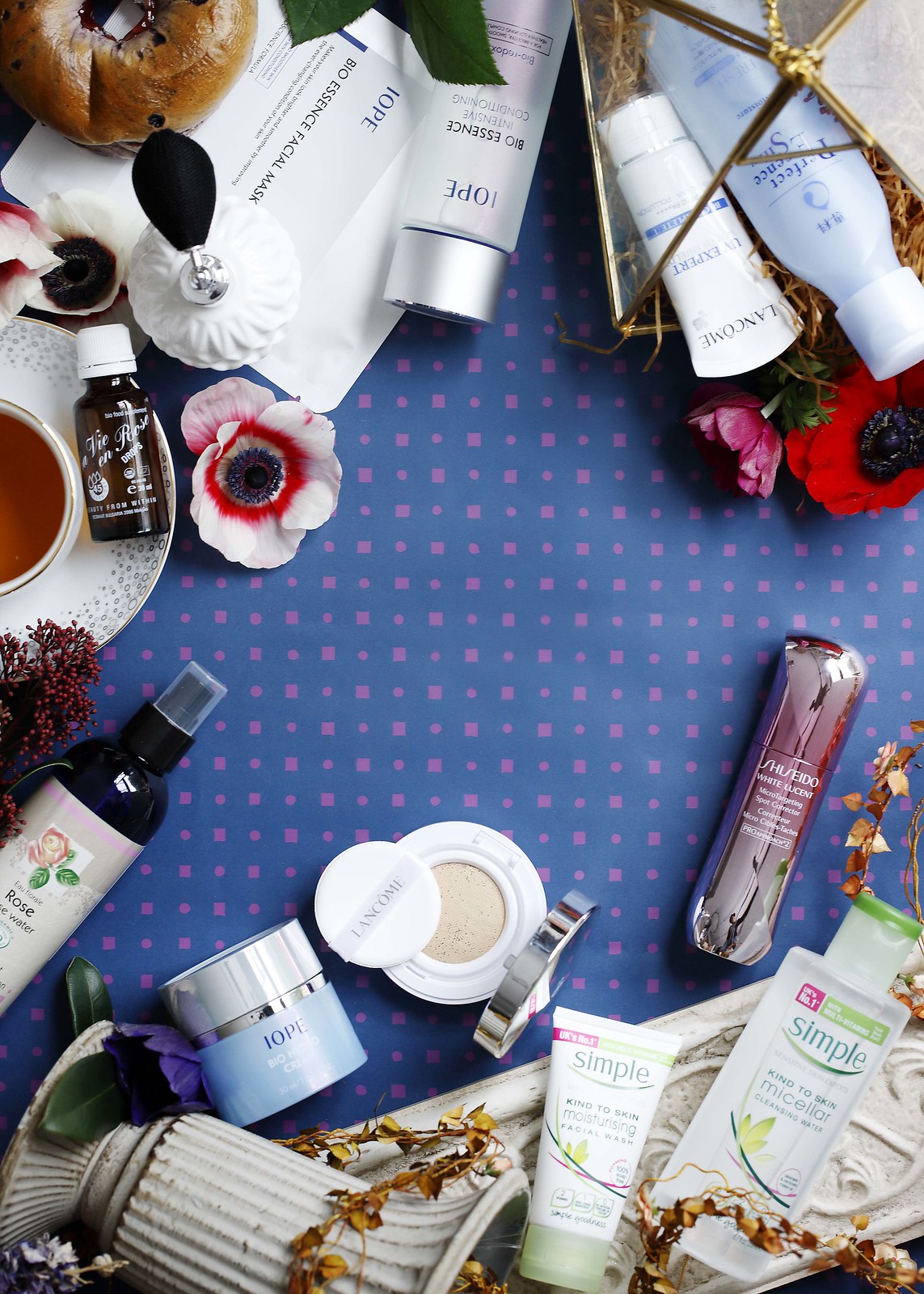The image features an artfully arranged collection of beauty products displayed on a blue surface adorned with small purple icons in the shapes of squares and circles. The products, meticulously arranged, include a variety of brands and items. In the bottom right corner, clear bottles with green tops from the brand "Simple" are visible. Nearby, products from Lancome and Shiseido are also present. On the left side, there's a black bottle labeled "Rose" and several items from the brand "Iope."

Among these cosmetics, additional objects add to the aesthetic. Stone vases with yellow vines, green leaves, a teacup and saucer filled with tea, and a mix of white, red, and pink flowers are interspersed throughout the arrangement. A portion of a pumpkin is also visible, contributing to the natural theme. A golden box containing yarn is included, along with a white perfume bottle with a black atomizer. Underneath some products, a letter can be seen, completing the artistic display.